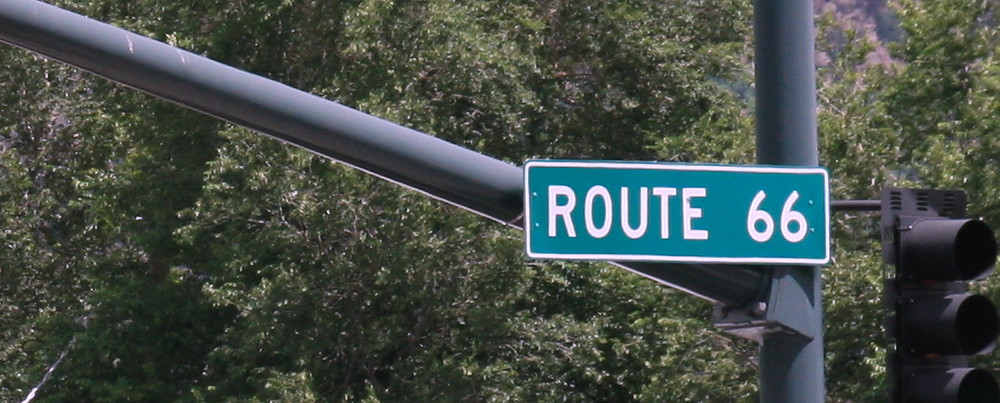In this image, we see a traffic light mounted on a dark green pole. The traffic light itself is black, although it's unclear which light is currently activated. The pole, which may be supporting another light, also displays a green sign with white letters that read "Route 66." The sign is bordered in white. The background is filled with dense trees and foliage, adding a natural contrast to the urban elements. Towards the upper right corner of the image, there appears to be a hill or mountain in the distance, contributing to the scenic backdrop. The pole extends vertically upwards before bending horizontally to the left, supporting additional infrastructure.